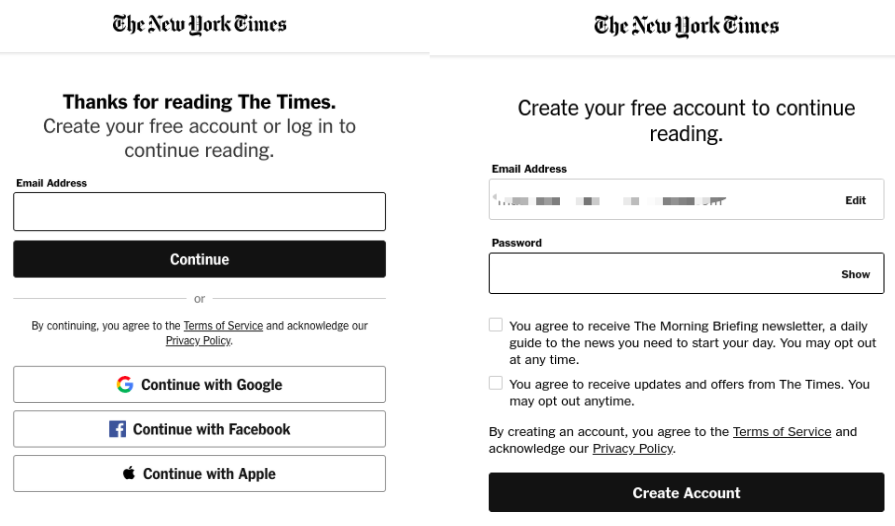This image is a detailed screenshot of a New York Times webpage prompting users to create a free account or log in to continue reading. At the top of the page, "The New York Times" is prominently displayed as the website's header. On the left side of the screenshot, there is a message thanking the reader for visiting and instructing them to either create a free account or log in. It lists options for account creation, including entering an email address or using third-party services like Google, Facebook, and Apple to continue.

To the right, detailed text outlines the steps to create an account. Users are prompted to input their email address and a password (with an option to show the password). There are checkboxes for agreeing to receive the morning briefing newsletter and updates or offers from The Times, both of which allow users to opt out later if they choose. A black rectangle at the bottom of this section contains white text that reads "Create Account."

This image is entirely text-based with no photographic elements, no people, animals, plants, or buildings present. The section where users would enter their email address is blurred out for privacy.